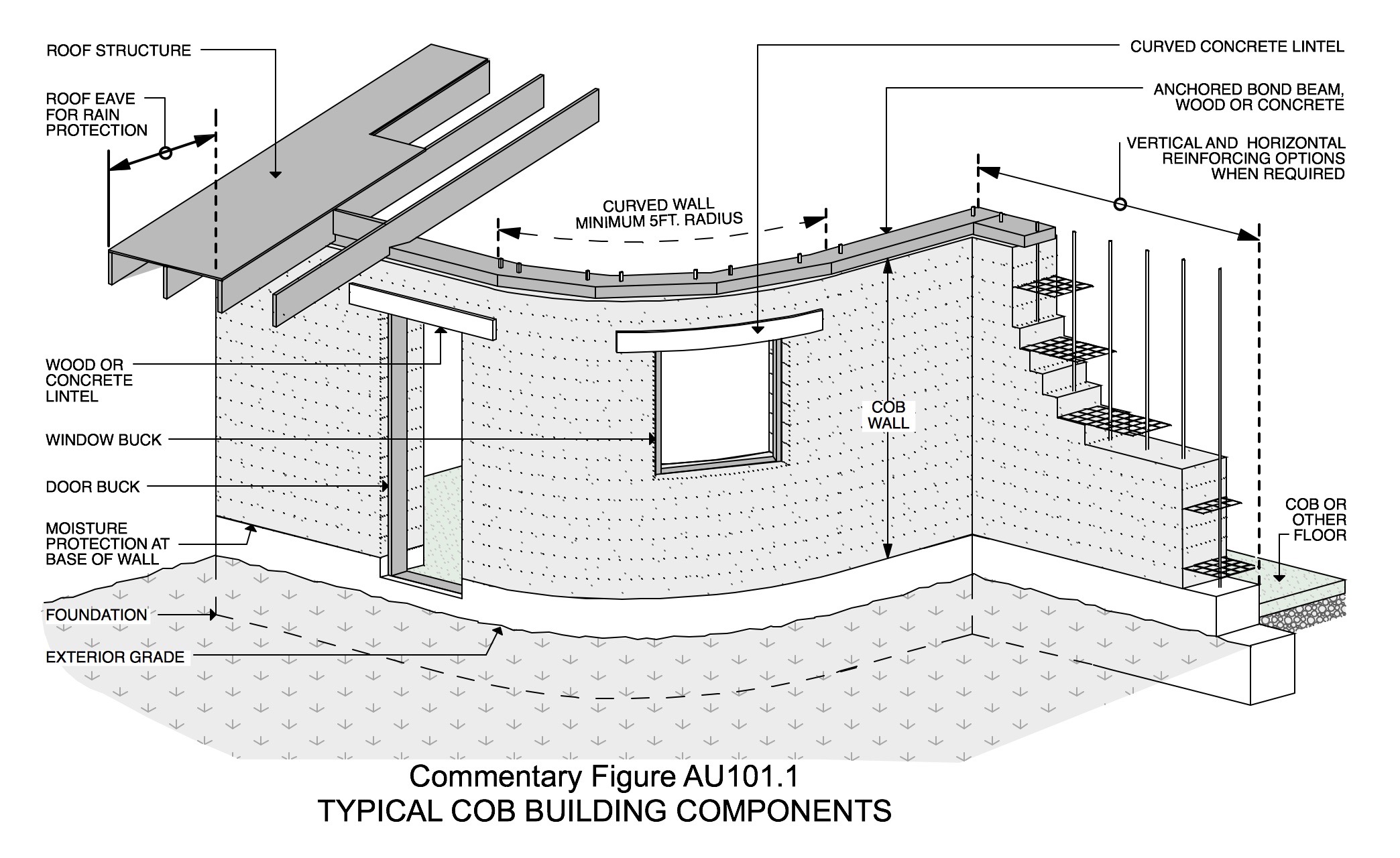The image depicts a detailed architectural blueprint or diagram of a building section, primarily in black, white, and shades of gray with some green accents. A rounded wall is prominently featured, showing both its interior and exterior components. The spherical-shaped wall includes a window and a door, with additional elements like staircases and flooring. Different areas are meticulously labeled with lines and arrows pointing to specific parts: for instance, the roof is divided into sections such as "roof structure" and "roof eave for rain protection," while the door border is marked as "door bark," and the window's edge as "window bark." The diagram also highlights structural elements like a "concrete lintel" above the window, an "anchored bond beam" at the top, and "moisture protection at the base of the wall." The layered components of the wall, including types of poles and gratings, are identified. The bottom portion of the blueprint features the title in black print: "Commentary Space Figure AU101.1 Typical COB Building Components." The drawing provides a comprehensive overview of both horizontal and vertical reinforcing options and structural materials used within the depicted building section.